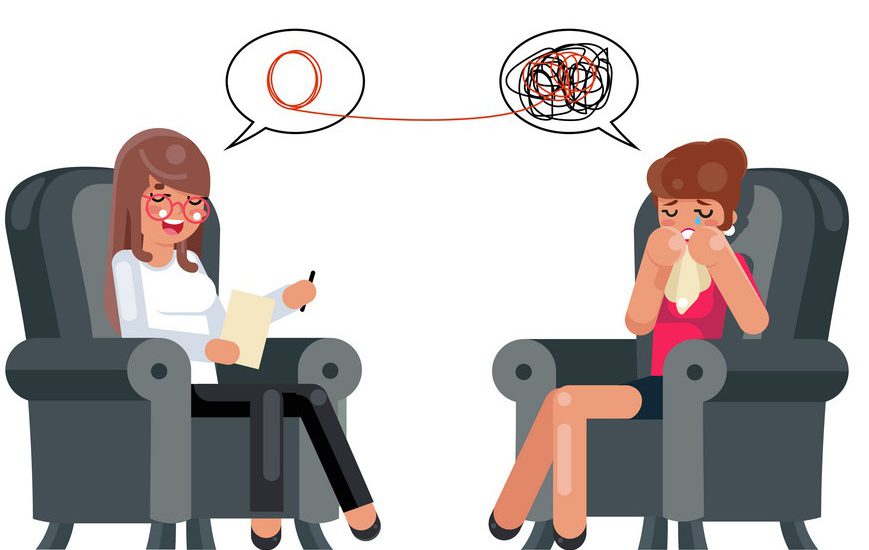The image is an illustration featuring two women seated on dark grey couches with armrests. The left-hand woman, with long dark brown hair and red glasses, is wearing a long-sleeve white top, black trousers, and black shoes. She holds a piece of paper in one hand and a black pen in the other, appearing to read something aloud with a slight smile. A speech bubble above her head contains a red, spiral thread-like structure, symbolizing coherent speech. The right-hand woman, with brown hair tied up, is dressed in a short-sleeve hot pink top and black shorts. She is crying, holding a white handkerchief to wipe her blue tears, and her speech bubble is filled with a garbled pattern of black and orange scribbles, indicative of emotional distress. The background is white, emphasizing the contrasting emotions of the two characters in this cartoon-like setting.